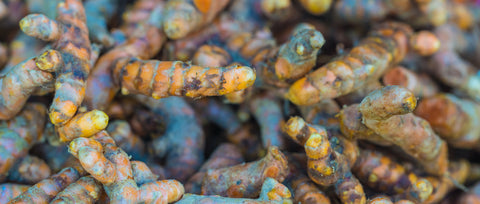This close-up photograph captures a chaotic mound of long, cylindrical objects with varying colors and textures that evoke both organic and inorganic imagery. Dominated by bright yellows, bold oranges, and hints of blues, greens, purples, and browns, each element is covered in dirt and features striations along their lengths. With an unclear context, the objects resemble a mix of finger-length roots, worms, and even snails, creating a perplexing scene. Despite the absence of a clear size reference, dozens of these colorful, dirt-encrusted items mesh together in a small, horizontal frame. Some appear to have small dark spots that could be mistaken for eyes, adding to the eerie, almost alien quality of the pile.